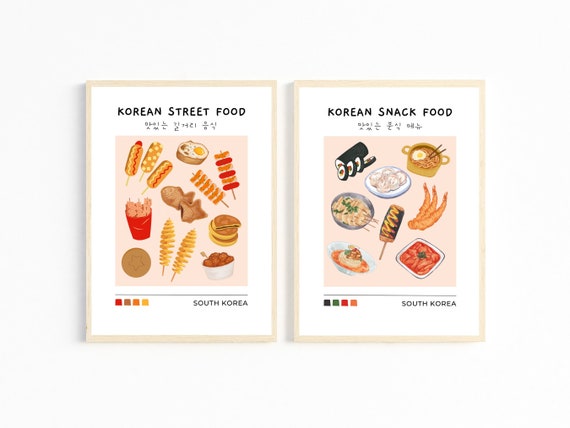The image features two framed prints set against a white background. Each print, encased in light brown wooden frames and resembling an 11 by 14 style, showcases a detailed comparison of Korean culinary delights. Both frames are in a vertical, portrait layout.

The print on the left is titled "Korean Street Food" in bold, black, all caps at the top. Directly beneath, a line of small Asian lettering likely spells out the same phrase in Korean. Encased within the frame, a beige background sets off colorful, cartoonish illustrations of various street foods, including corn dogs, shish kebabs, French fries, a sandwich, and a bowl of tater tots. Additional design elements include four colored squares—red, brown, orange, and yellow—along the lower left side. The bottom right corner of the print bears the label "South Korea."

Mirroring the first, the print on the right is labeled "Korean Snack Food" in the same bold, black, all caps text at the top, likewise followed by smaller Asian lettering. The central illustrations, also set against a beige background, depict an assortment of snack foods, such as sushi, dumplings, shrimp, ramen, and items that resemble a bento box and something in red sauce. This print also features a series of four darker shaded colors along the left side. Like its counterpart, it concludes with "South Korea" printed in the bottom right corner.

Overall, the harmonious design and parallel structure of the prints offer a vivid, illustrated guide to Korean street and snack foods, bringing the vibrant culinary culture to life.